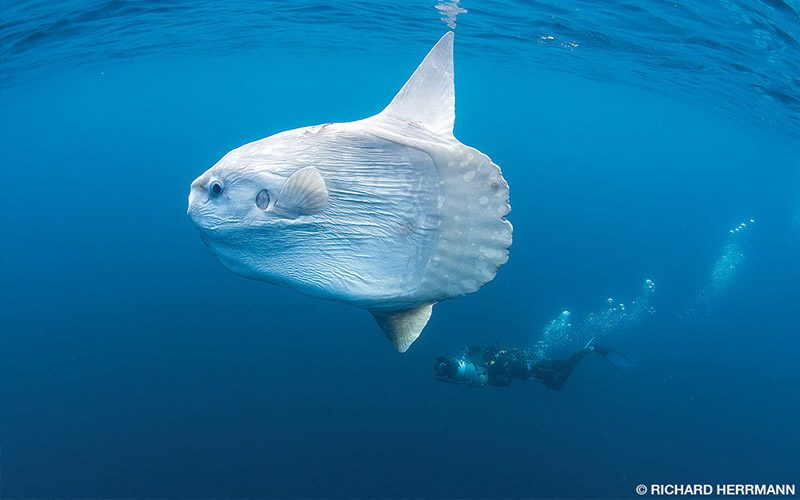In this underwater photograph, the viewer's eye is immediately drawn to a large, beautifully translucent white fish with strikingly prominent white fins and gills. Its intricately scaled tail fans out like seashells, and its dark blue eye adds a compelling detail to its gentle, ghostly appearance. The fish is positioned towards the top-left of the image, seemingly gliding near the surface where light from above still penetrates the depths, creating varying shades of blue that grow darker towards the bottom of the frame. Beneath and slightly to the right of the fish, a scuba diver, clad in a standard black diving suit with flippers and an oxygen tank, is likely photographing the majestic creature, evidenced by the bubbles trailing behind him. Interestingly, the lower right corner displays the text "Richard Herman," suggesting the photographer’s signature or copyright mark, grounding the viewer in the scene's authenticity. The ocean setting, with its vibrant blues and subtle grays, encapsulates a serene yet dynamic underwater world, capturing an extraordinary moment of coexistence between human and marine life.